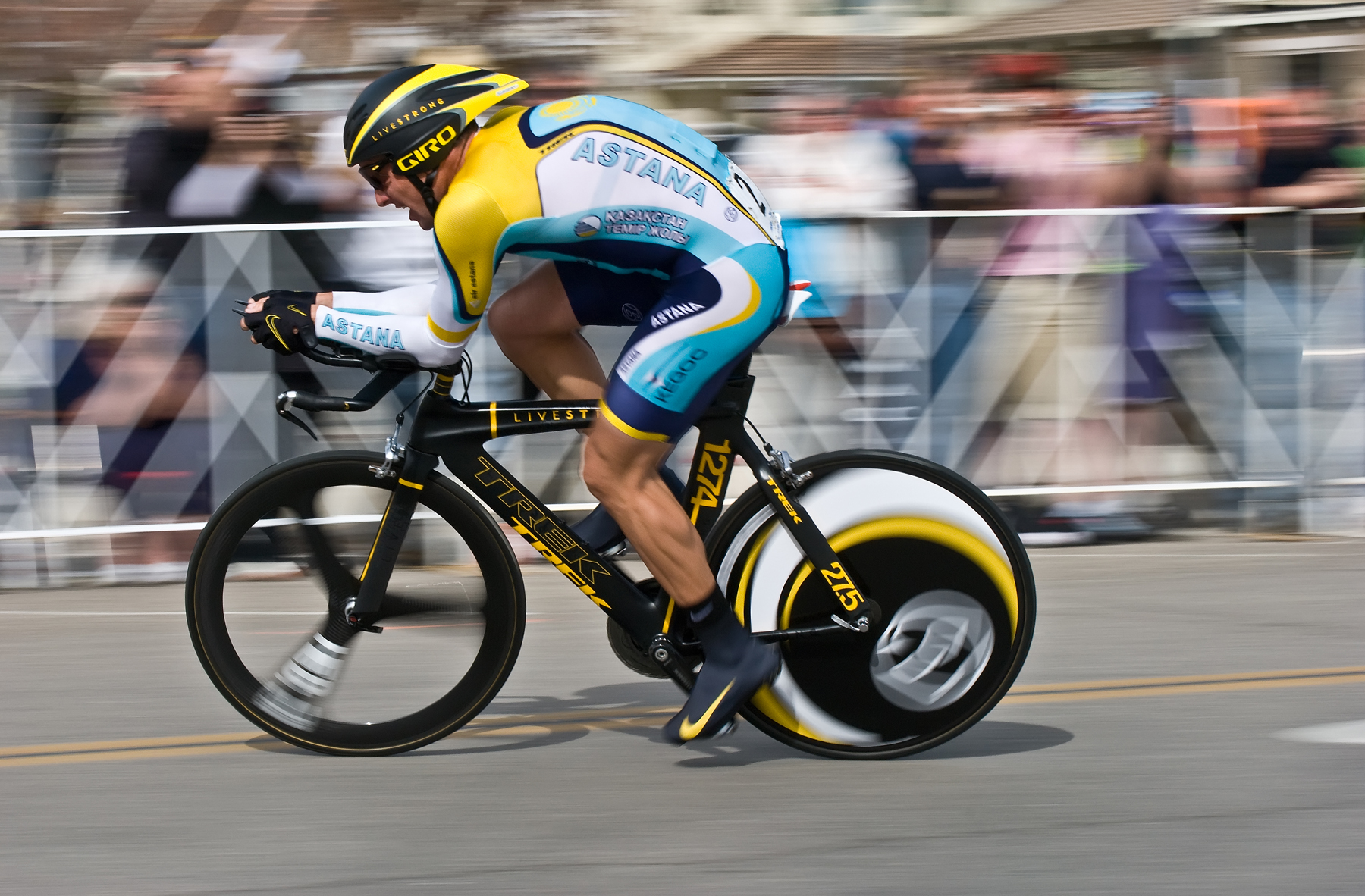In this image, a male cyclist, dressed in a tight race outfit, is actively participating in a bike race. His sleek, aerodynamic jersey prominently features the name "Astana" in white and blue letters against a background of yellow, light blue, and white. He's equipped with a black bike that has yellow lettering reading "Trek" on the frame, and it's paired with a solid back wheel and a three-spoked front wheel. The rider's outfit is complemented by yellow and black Nike racing shoes and a pointy black and yellow helmet with the label "Giro" in yellow. The road beneath him is grey, marked with white and yellow lines. Behind a white fence, there’s a blurred crowd of spectators, emphasizing the rider's speed and the motion of the race.